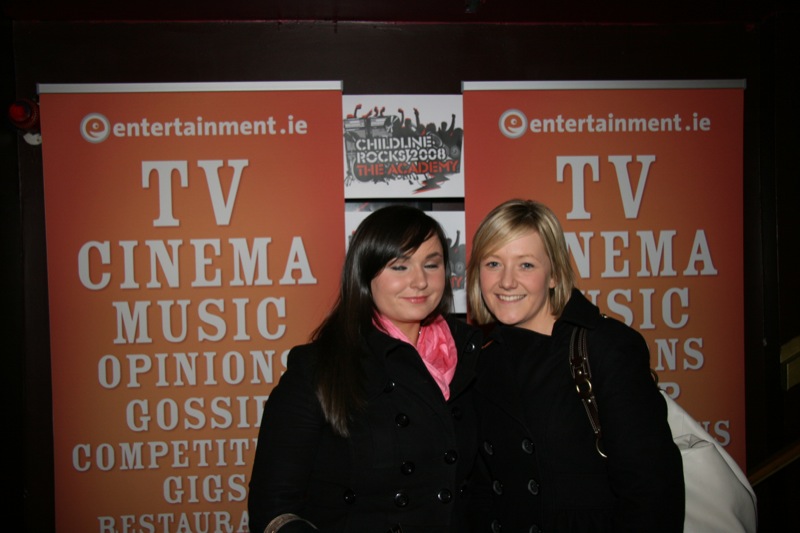In the photo, two women, likely in their 20s or 30s, are posing at an event in front of two identical pull-up banners. The banners have an orange background with white text that includes words such as "TV," "Cinema," "Music," "Opinions," "Gossip," "Competition," "Gigs," and "Restaurants." The top of the banners features the logo "entertainment.ie." Between the banners, there's a smaller sign that reads "Childline Rocks 2008 The Academy," against a black wall.

The woman on the left has shoulder-length black hair and is wearing a long black jacket with visible buttons and a pink scarf peeking out from underneath. She is smiling with her eyes closed. The woman on the right has dirty blonde hair and is also dressed in a long black jacket with buttons, accessorized with a large purse on her left shoulder. She is smiling at the camera.